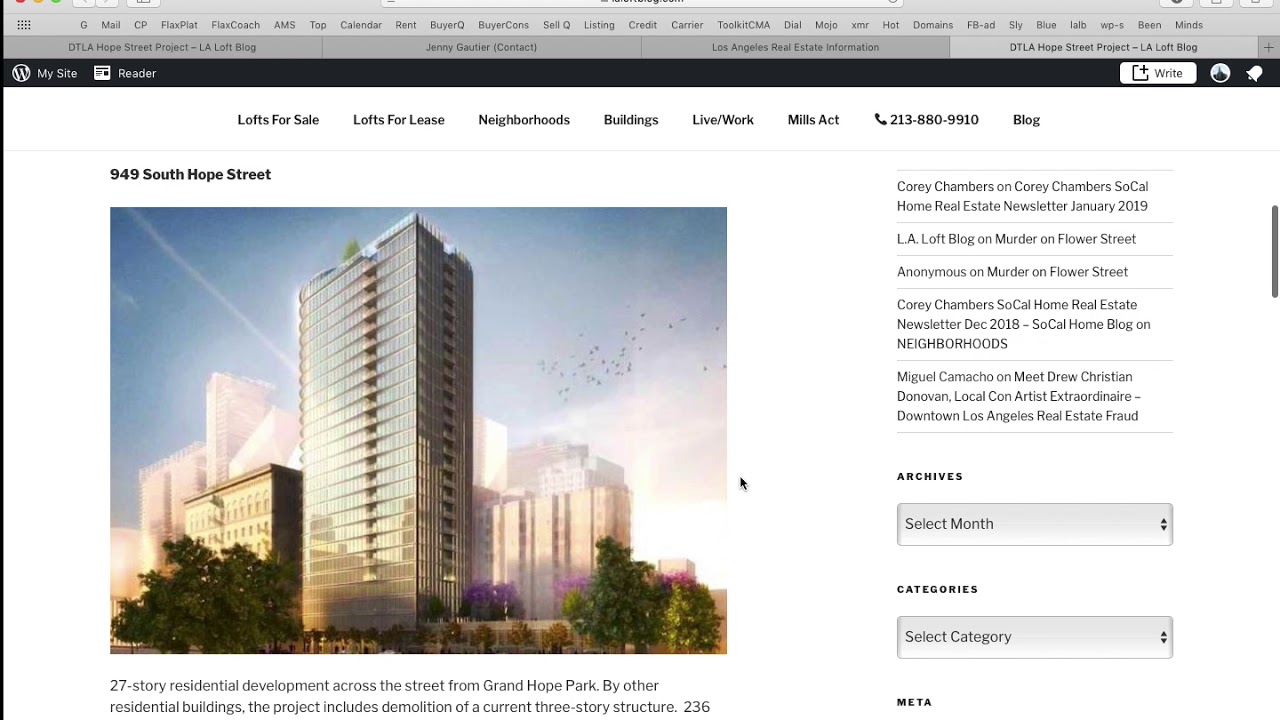This image appears to be a screenshot of a computer screen displaying a website. The top section of the image features a gray background with a horizontal navigation bar listing various menu items such as "Mail," "CP," "AMS," "Top," "Calendar," and several others extending to the right. Below this navigation bar, there is a darker gray line containing additional written elements, followed by a black bar with white text that reads, "My Site, Reader."

Further down, the background transitions to white, indicating the main content area of the website. The top of this section offers several navigation options: "Lofts for Sale," "Lofts for Lease," "Neighborhoods," "Buildings," "Live/Work," "Mills Act," along with a contact phone number and a link to a blog. 

Central within the white background is an image of a high-rise apartment building. Directly above the image, the address "949 South Hope Street" is prominently displayed. Below the building's picture, some brief information about the building is provided. To the right of this description, there is a detailed list of amenities or features associated with the building.